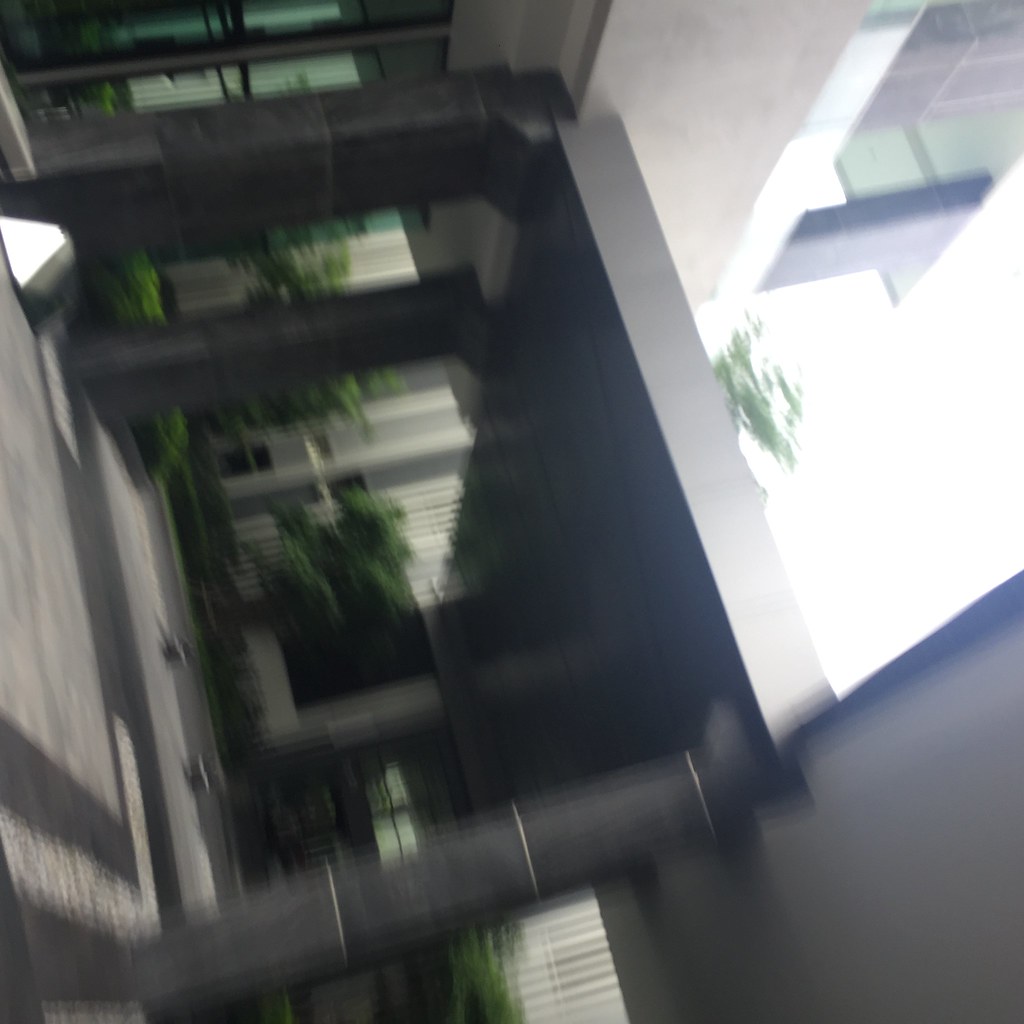A modern building stands tall, primarily constructed of glass panels with some cement elements, giving it a sleek and contemporary appearance. The image appears to have been rotated 90 degrees to the right, creating an unconventional perspective. In front of the building, a breezeway supported by several poles provides a covered walkway. The daytime sky, though not particularly bright, adds a serene backdrop to the scene. A few trees and bushes are visible, adding a touch of greenery to the urban landscape. The building itself maintains a significant height and extends well to both the left and right, emphasizing its impressive scale.